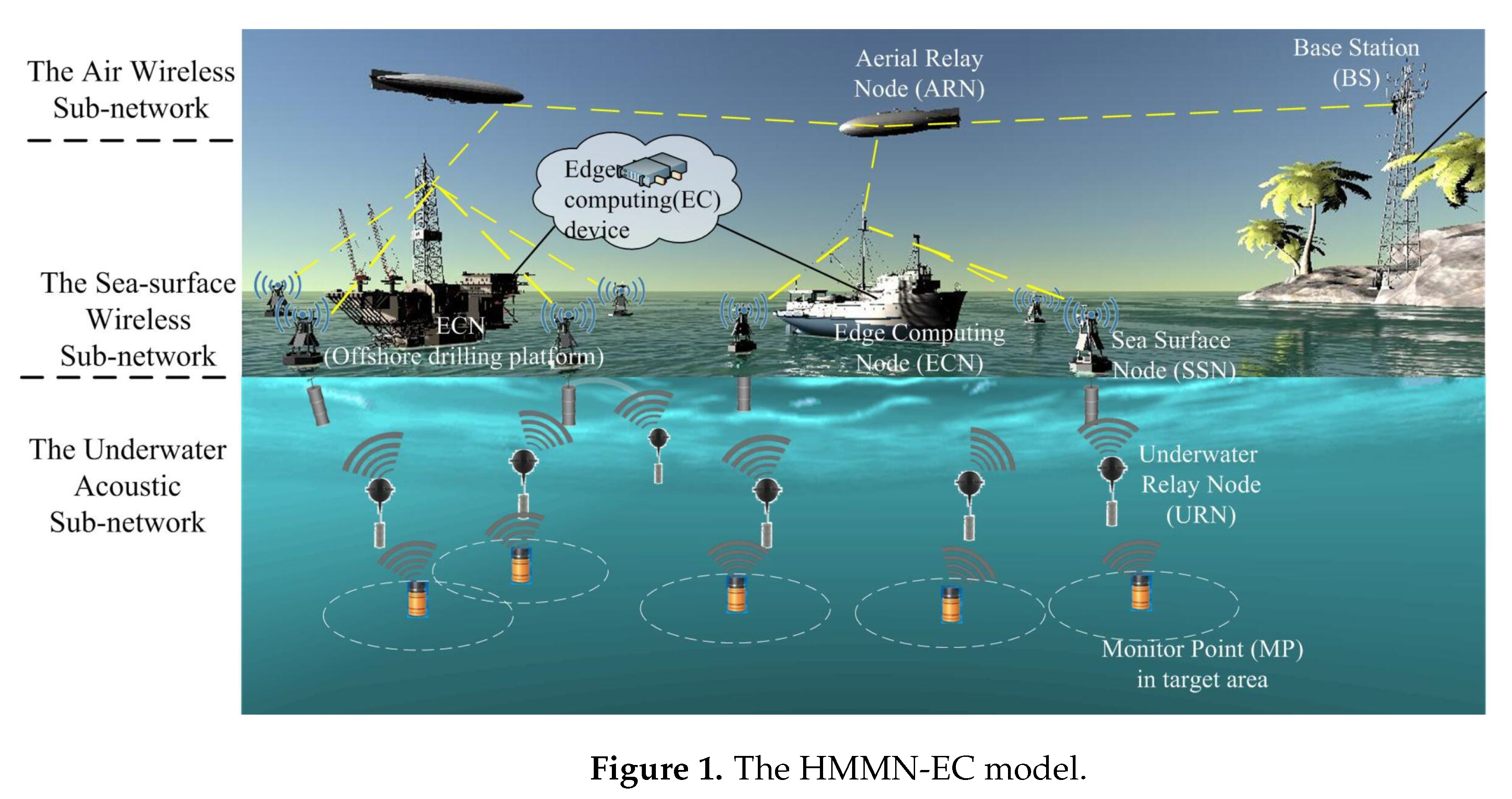The image is a detailed 3D-rendered, landscape-format diagram labeled "Figure 1, the HMMN-EC model," which appears to illustrate a complex communications network, possibly for military purposes. The diagram is divided into three distinct sections: the Air Wireless Subnetwork at the top, the Sea Surface Wireless Subnetwork in the middle, and the Underwater Acoustic Subnetwork at the bottom. The upper section features dirigibles and drone-like structures in the air, receiving and transmitting radio waves. The middle section shows several ships on the water's surface. The right side of the image displays an island characterized by large boulders, palm trees, and a radio tower. The bottom section provides a cutaway view of the underwater environment, revealing labeled elements such as Underwater Relay Nodes (URN) and Monitor Points (MP). The entire illustration is annotated with labels and arrows, indicating complex interactions among the air, surface, and underwater elements.